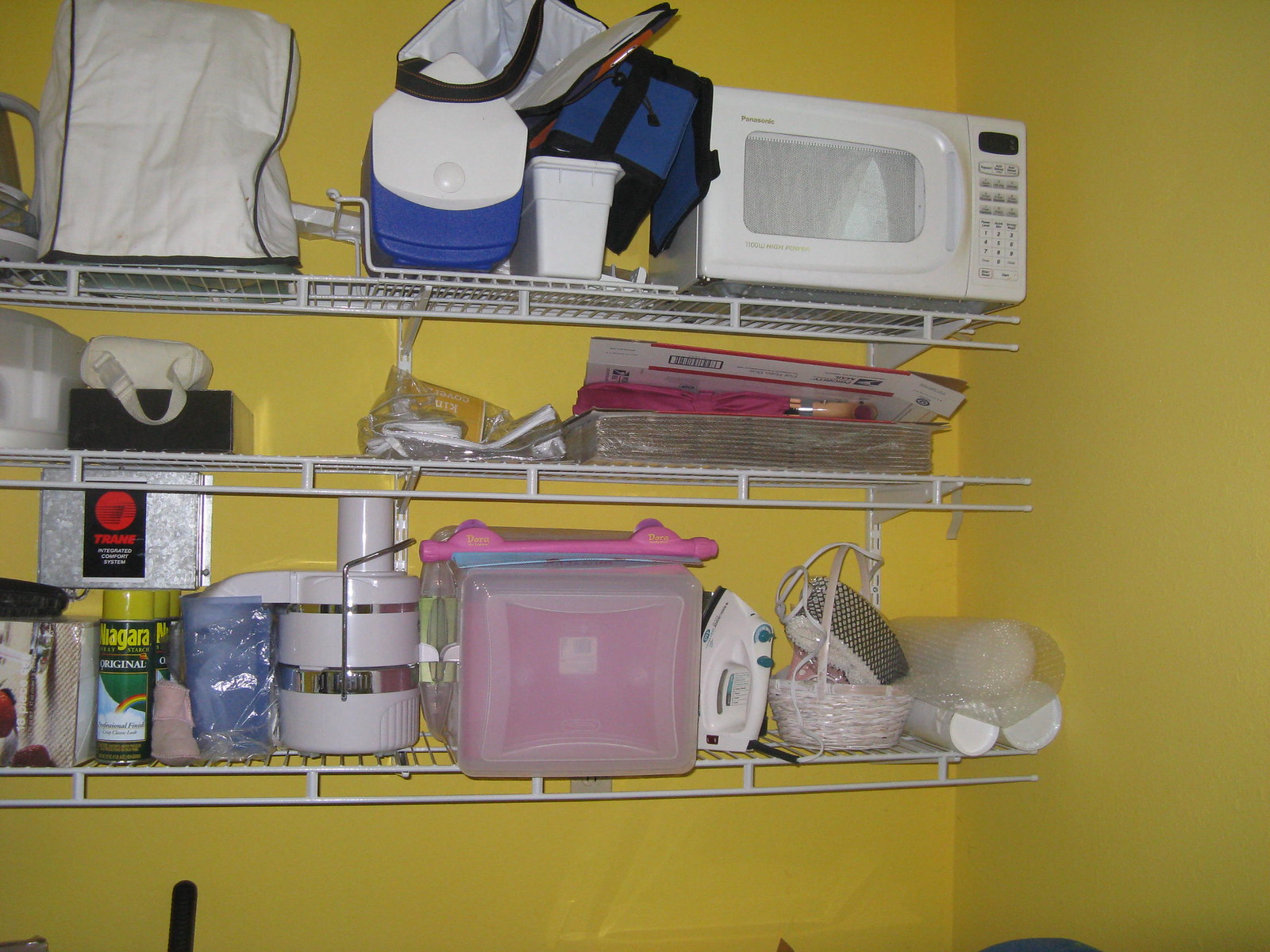This photograph showcases three white metal wire shelves mounted on yellow-painted walls. The shelves are supported by white angle holders and attached to vertical metal rails, giving the setup a structured appearance suitable for a laundry or storage room. Each shelf is utilized differently across three levels: 

- The top shelf holds a white microwave oven and several bags likely containing ice or frozen food.
- The middle shelf contains various flat items.
- The bottom shelf is stocked with cans of paint, parts of kitchen appliances, plastic boxes, an electric iron, baskets, and rolls of paper cups.

The overall scene depicts a well-organized but functional storage solution within a household setting.